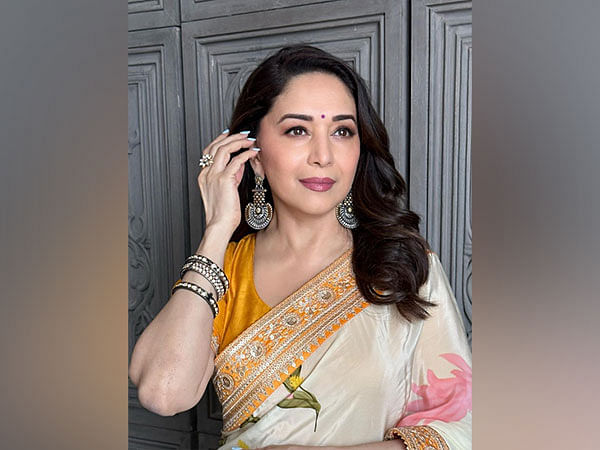The photograph features an Indian woman with long, dark, curly hair adorned with a red bindi on her forehead. She is dressed in a traditional Indian outfit, consisting of an orange dress with a white floral shawl that highlights intricate orange and silver embroidery around the neckline and cuffs. She accessorizes with silver dangly chandelier earrings, black and rhinestone bangle bracelets, and a flower ring on her right hand, with her fingernails painted blue. Her makeup includes pink lipstick, adding a touch of vibrancy to her visage. The surroundings include a gray wall and a wooden cabinet with carvings that complement the overall color scheme of the image. The intricate details in her attire and accessories, along with the backdrop, suggest a blend of cultural richness and aesthetic appeal.